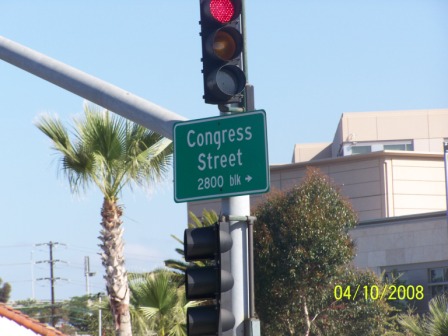A vivid street scene captured on April 10th, 2008, featuring a simple street sign for Congress Street. The street sign displays "Congress Street" in bold white text set against a classic green background. Positioned just below a stoplight glowing red, the sign stands prominently in the shot. In the backdrop, there is a charming palm tree, adding a touch of tropical flair, alongside a pristine white building that contributes to the urban landscape. The bright blue sky and the clear lighting indicate that the photograph was taken in the middle of the day, highlighting the pleasant weather and the tranquility of the moment.